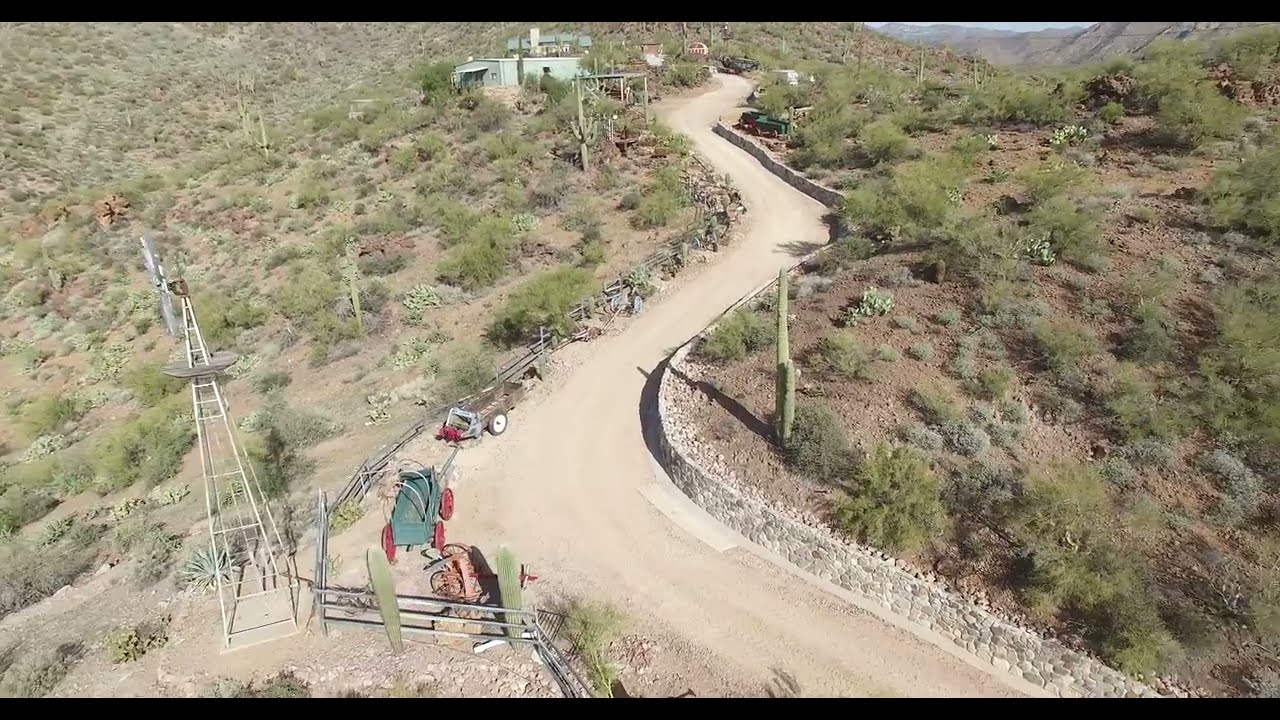The photograph depicts a green hillside adorned with patches of lush grass, bushes, hedges, and dense foliage. A long, winding dirt road snakes along the hill's crest, leading up to a cluster of buildings nestled amidst the verdant landscape. In the foreground, tractors and trailers are lined up beside a towering windmill, near a split rail fence and a stone wall that runs parallel to the road. Scattered around are old covered wagons and antique farm equipment, including a green wagon with red wheels and an old manure wagon. Among the buildings, notable structures include a green warehouse, possibly a small power plant, along with other green and white-roofed buildings. The entire scene is framed by distant mountains and hills, enhancing the picturesque, well-maintained rural setting.